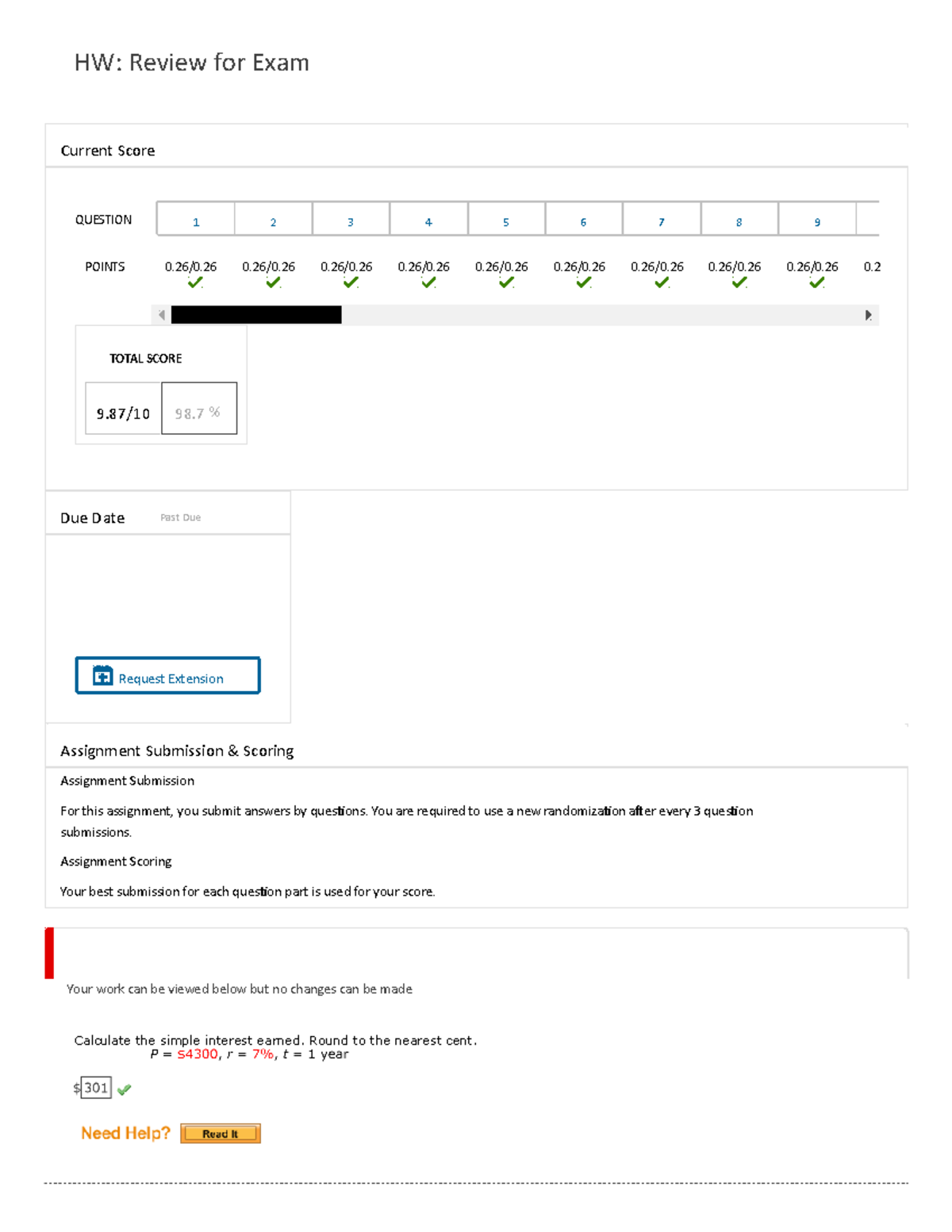Here is the cleaned-up and detailed caption:

---

The page displayed is an exam review interface presumably used by tutors for assessing students post-exam. The heading reads, "HW: Review for Exam." Below, the current score section is visible, showing a total score of 9.87 out of 10. The assessment comprises nine questions, each marked with a tick indicating completion. The due date field remains empty, suggesting it hasn’t been set yet. 

Users have a few actionable options, including a "Request Extension" button and an "Assignment Submission and Scoring" button. The interface requires answer submissions to be broken down by question, with a new randomization implemented after every three questions submitted. While this system is unfamiliar, it is likely associated with university or college coursework. 

At the bottom of the page, a prominent yellow button labeled "Need Help? Read It" is available for additional assistance.

---

This caption provides a comprehensive and structured overview of the interface, suitable for those unfamiliar with its function.